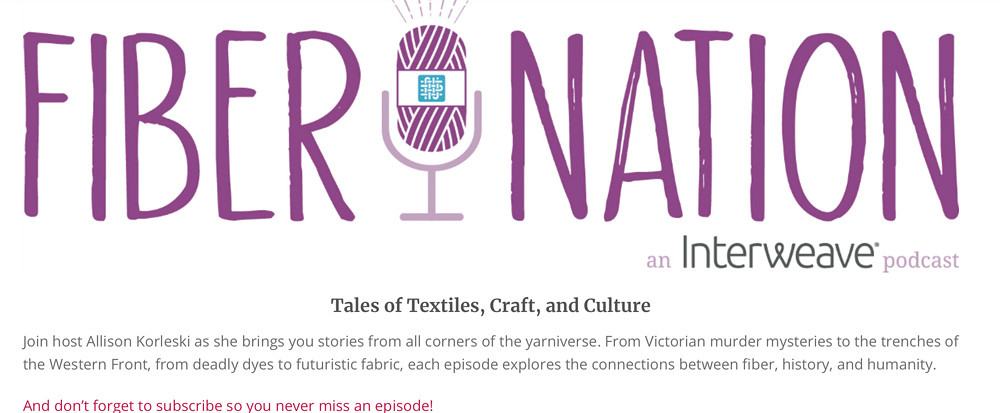Promotional image for the podcast "Fiber Nation," with the title prominently displayed in purple. At the center, a microphone separates the words "Fiber" and "Nation." Beneath the logo, the tagline reads, "Tales of Textiles, Craft, and Culture." Viewers are invited to join host Alison Koleski as she delves into captivating stories from the far corners of the Yarniverse, covering topics like Victorian murder mysteries, World War I trenches, deadly dyes, and futuristic fabrics. Each episode examines the deep connections between fiber, history, and humanity. In bold red text, the promotion reminds viewers, "Don't forget to subscribe so you never miss an episode." This podcast is brought to you by Interweave.